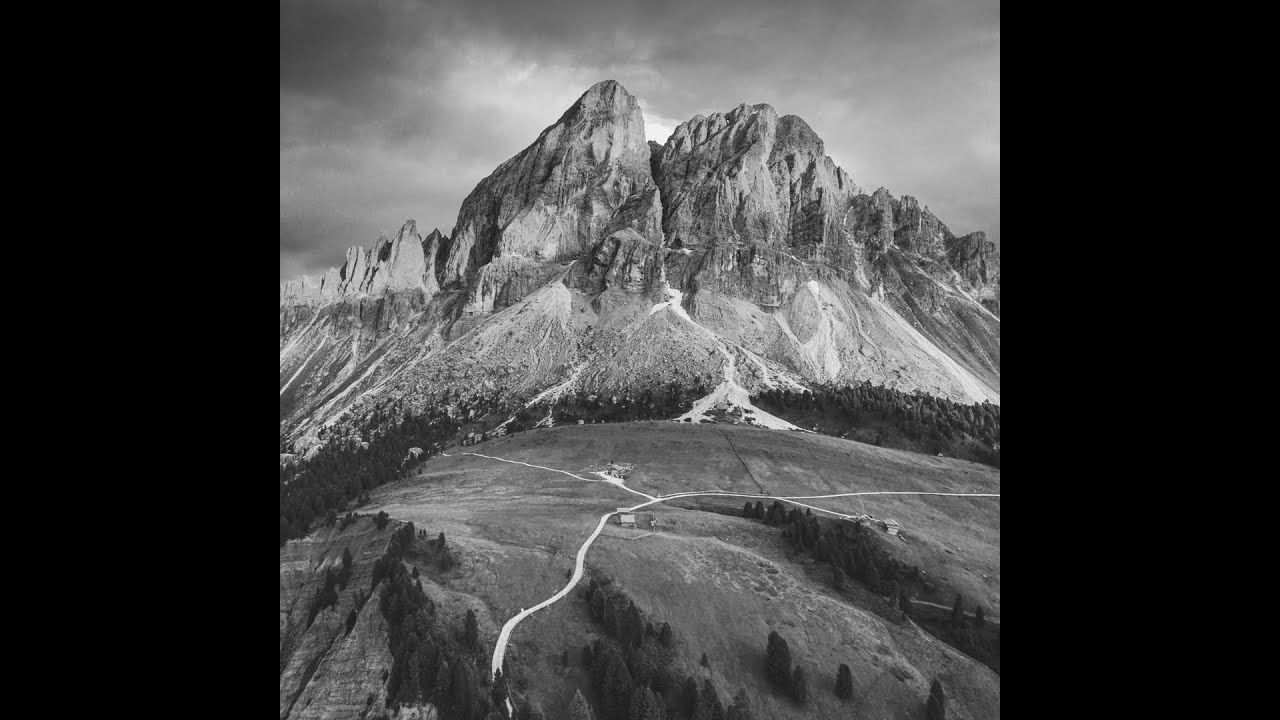This black-and-white photograph, presented in a square format with blank black spaces on the left and right to create a widescreen effect, captures a serene yet dramatic landscape. The scene features a grass-covered hill foreground, with intersecting roads leading to a small house and clumps of pine trees scattered around the lower elevations. Dominating the background, a towering rocky mountain range rises abruptly, displaying jagged, vertical rock formations. A white line marking a central road ascends the hill, leading up to a plateau. The sky above is densely clouded, with subtle light breaking through, enhancing the moody grayscale of the image.